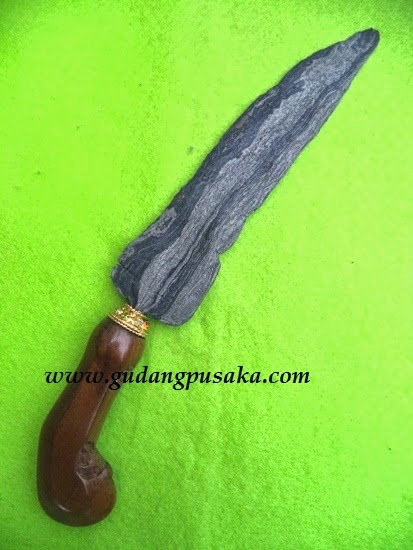The image is a small, vertical, rectangular photograph featuring a knife set against a bright green background. The knife, positioned diagonally from the lower left to the upper right corner, appears to blend elements from different eras. The blade looks like it is roughly made out of stone, evoking an ancient, Stone Age aesthetic. In contrast, the handle is a polished, nicely carved wooden piece, likely mahogany, suggesting craftsmanship from a much later period, potentially the 17th or 18th century. The handle is curved at the bottom and attached to the blade with a gold fitting. The knife also seems to be partially encased in a scabbard, enhancing the historical feel. The background, possibly a green cloth or lime green surface, complements the earthy tones of the knife. Additionally, there's a visible web address, www.gudangpusaka.com, indicating a platform where this image can be viewed. Overall, the image juxtaposes the crude, ancient blade with a refined, modern handle, creating a striking, artistic representation.